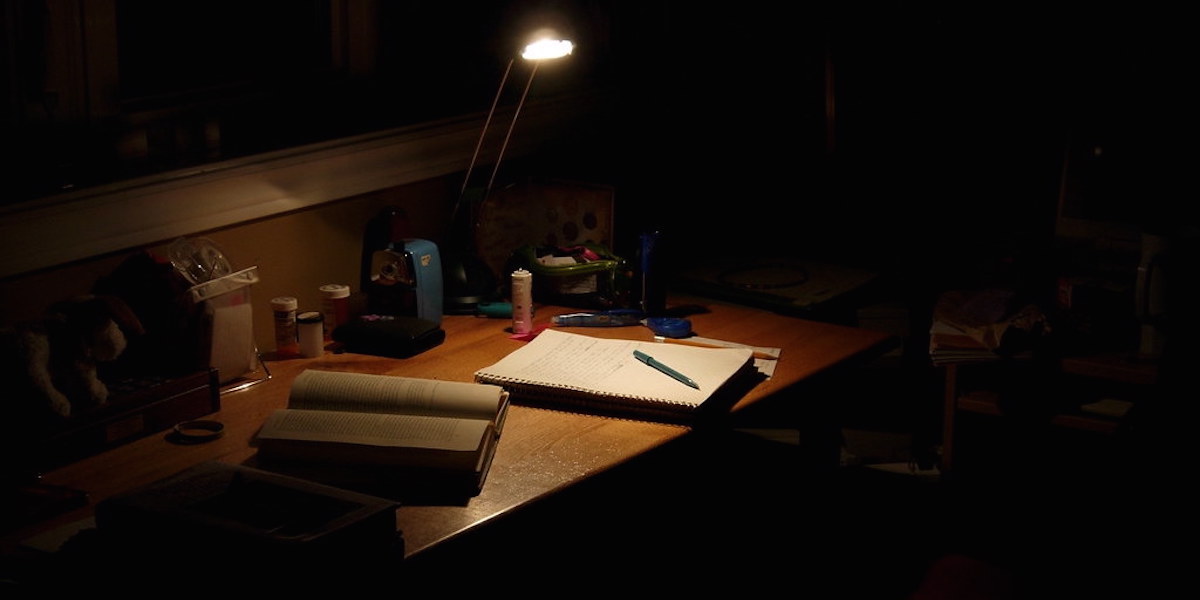This nighttime photograph captures a brown wooden desk illuminated solely by a single silver-colored desk light, creating a stark contrast against the otherwise dark room. The light, attached and positioned about a foot above the desk, casts a focused glow on a white spiral notebook with some writing on it and a pen resting atop. Just to the left of this notebook, an open book lays spread out, with another closed book barely visible in the shadows nearby. Various small containers, likely prescription bottles, are scattered towards the back of the desk. Positioned near the front of the notebook is a dark blue rectangular object, possibly a pencil sharpener. The desk is pressed against a wall with brown paint and features a white ledge that may be the base of a window. The objects and lighted area are clearly defined, while the edges of the image recede into darkness, emphasizing the solitude and focus of the workspace.